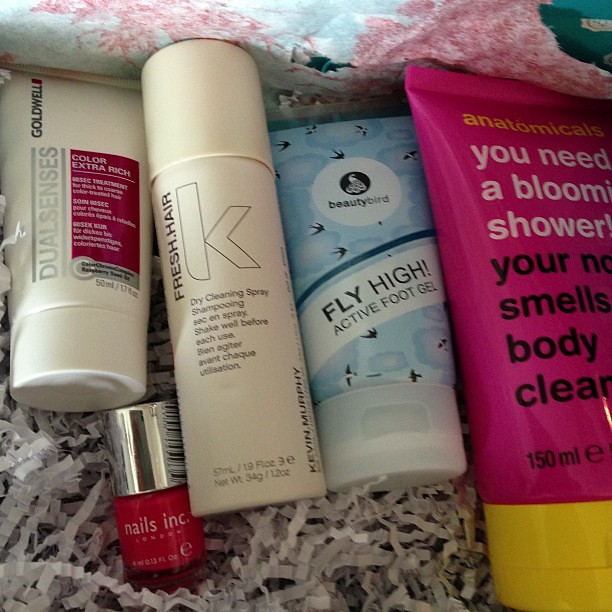This is a perfectly square image displaying a curated assortment of beauty care products arranged neatly in a white box filled with raffia stuffing and crinkled tissue paper. The box is set against a backdrop that appears to be a white tablecloth with a pink design. 

On the far right of the box, there's a bright pink tube with a yellow cap, branded by Anatomicals, with partially obscured white and black text that reads "you need a blooming shower" and "your smells body clean." To its immediate left is a blue and white tube labeled "Beauty Bird Fly High Active Foot Gel," embellished with flying bird graphics. Further left is a beige bottle that reads "Fresh Hair Dry Cleaning Spray Shampoo," advising users to shake well before use. 

At the very left edge is a white tube with a red rectangle that states "Goldwell Dual Senses Color Extra Rich," a type of hair treatment. Nestled just below this tube in the lower left corner is a small bottle of red nail polish with a silver cap, identified by the brand "Nails Inc."

Together, these five distinct beauty products are artfully displayed within the textured and protective filling, offering a visually pleasing and organized presentation.